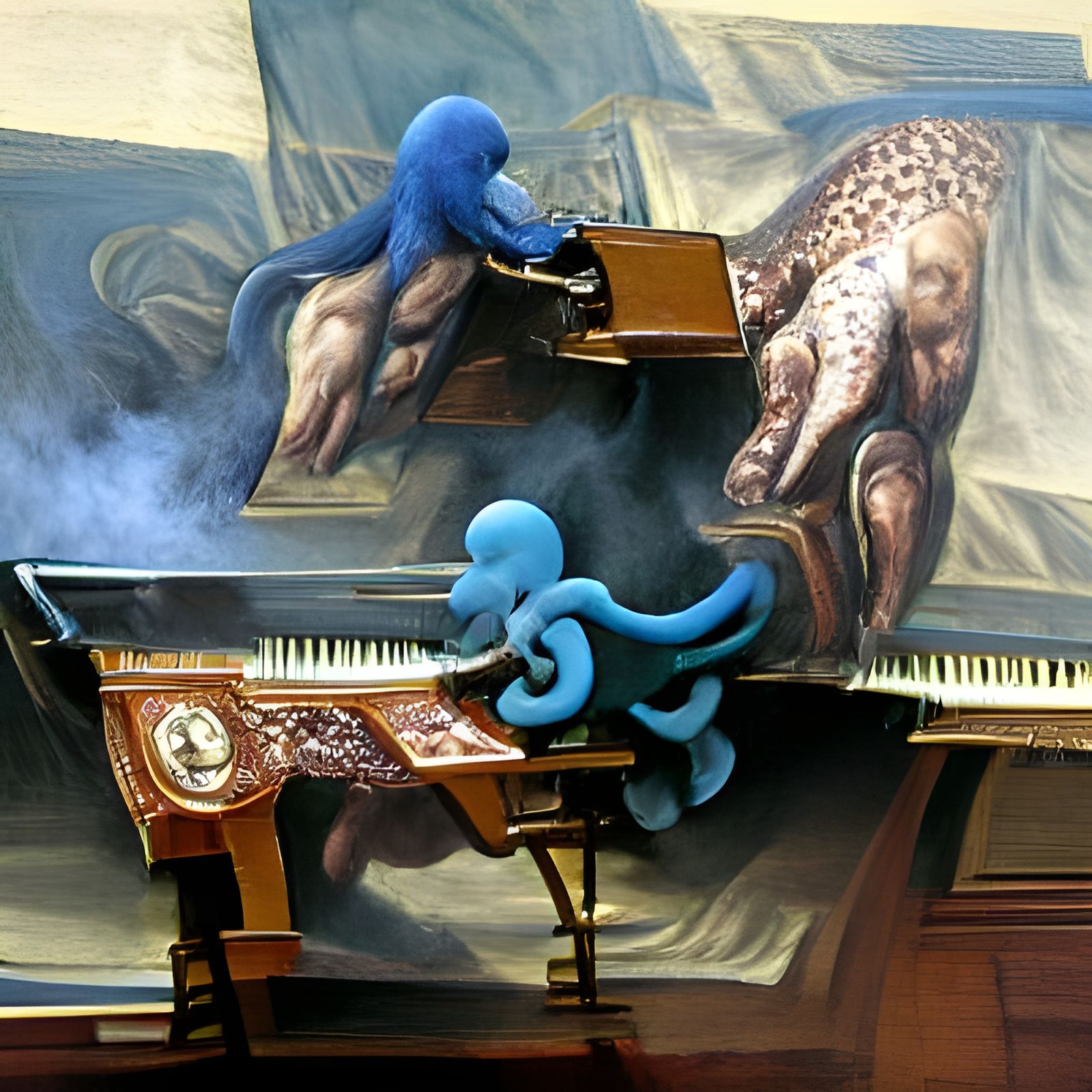This surrealistic painting, reminiscent of Salvador Dali’s style, features a black piano as its central element. The piano is set against a backdrop that evokes a wooden stage, where blue, animal-like figures appear to be playing it. The scene is highly abstract, with elements morphing into one another, creating a sense of fluidity and transformation. At the top of the painting, eagle and whale-like forms emerge, blending into a tan and brown figure that resembles a large chicken. Waves and intricate lines in hues of blue dominate parts of the composition, adding to the painting's musical and dreamlike quality. The artwork captures a dynamic and fantastical rhythm, emphasizing the surreal movement and blending of shapes and colors.